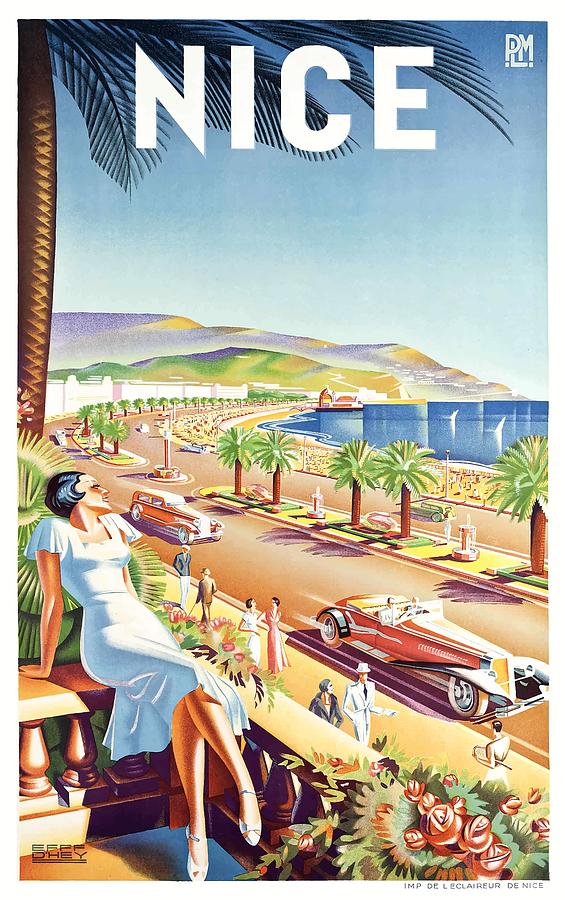The image is a stylized artwork, possibly the cover of a postcard, depicting a vibrant coastal city. Dominating the top of the image are bold white letters spelling "NICE," with the additional letters "P-L-M" overlapping in the upper right corner. The background features a striking blue sky and a mountain range in shades of gray, yellow, green, and dark blue, stretching across the entire width of the image. Below this, a sliver of dark blue ocean contrasts with the sandy outlines of the beach, where tiny figures or chairs are scattered.

A giant palm tree rises from the left side of the picture, its fronds reaching across the top. Towards the center, two vintage red cars—one a convertible, the other a regular car—are seen traveling down winding roads that curve towards the mountains. These roads are separated by a median filled with palm trees and fountains. Various people can be seen walking along the streets.

In the forefront on the left, a woman is prominently seated on a concrete railing with pillars, surrounded by roses. Her head is thrown back, revealing her short black hair, and she is dressed in a light blue summer dress that falls to her knees and has short sleeves. The woman completes her relaxed pose with crossed legs and sandals. There's also illegible smaller black text and some tiny French writing in the lower left corner of the image.